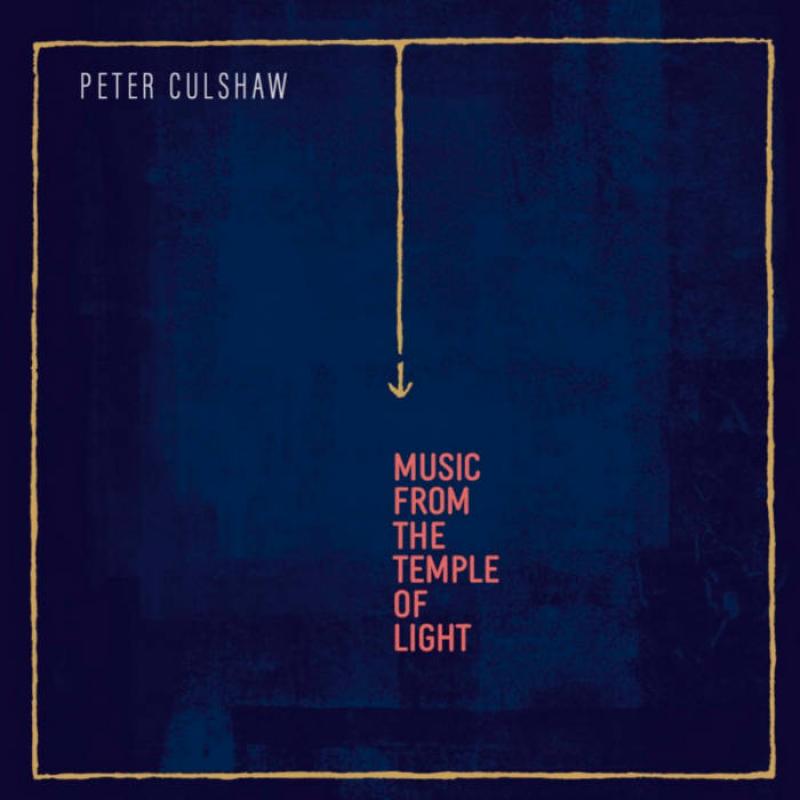The album cover features an intricate design composed mainly of color and text elements. The overall background is a spectrum of deep blues, blacks, and purples. Encasing the image is a yellow border. A striking yellow line, which transitions into a downward-facing arrow, runs from the top center towards the middle of the cover. At the top left corner, the artist's name, Peter Coleshaw, is prominently displayed in white text. Centrally positioned, the album title, "Music from the Temple of Light," is written in a vertically stacked fashion with each word placed directly beneath the previous one. The letters are an orange or salmon hue, drawing attention towards the center where the yellow arrow points. The cover's minimalist design focuses on text and simple geometric elements, creating a striking yet uncomplicated visual.